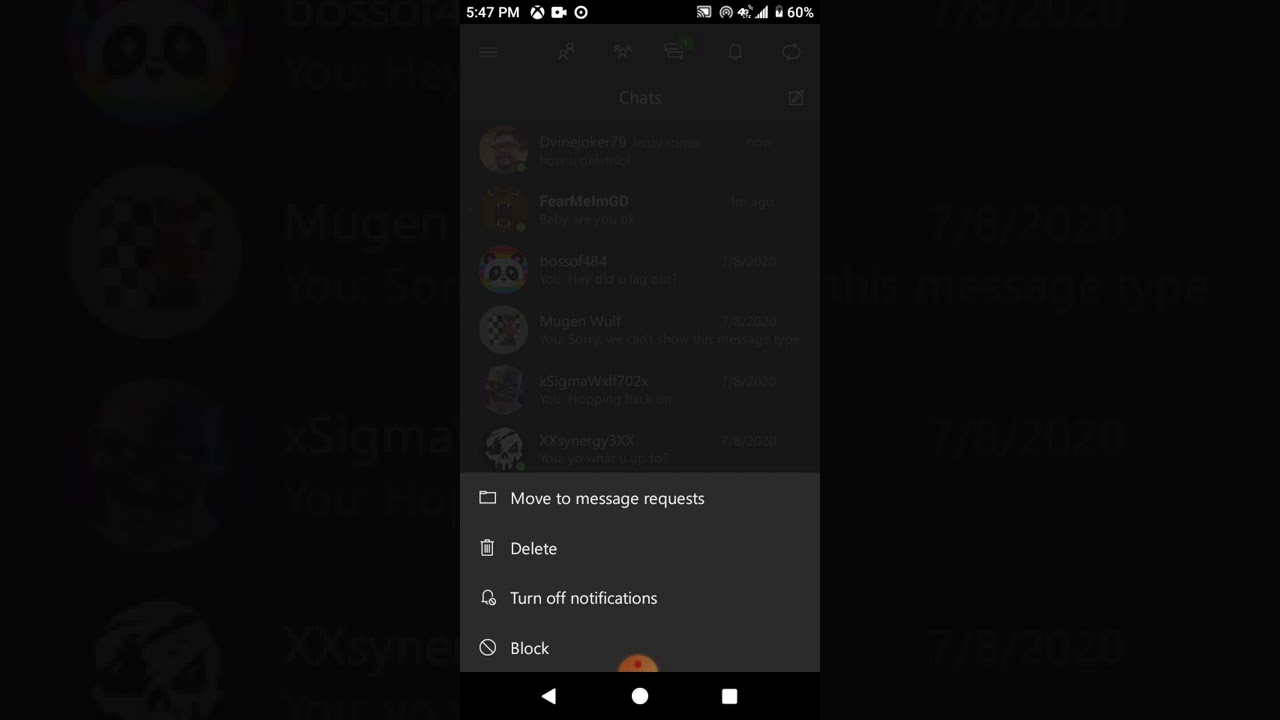The image showcases a screenshot prominently placed in the center of a blank background. In the top left corner of the screenshot, the device's current time is displayed as 5:47 p.m., alongside the Xbox icon. Moving to the top right corner, there are indicators for network signal strength and battery status, which shows the device is at 60% charge and currently charging.

Within the screenshot, several options are visible, including actions such as "move to message," "request," "delete," "turn off notifications," and "block." The screenshot also captures a chat interface featuring messages from "Divine Joker" among other participants.

At the bottom of the image, the standard navigation keys for an Android device are present: the back navigation key, the home key, and the recents app key.